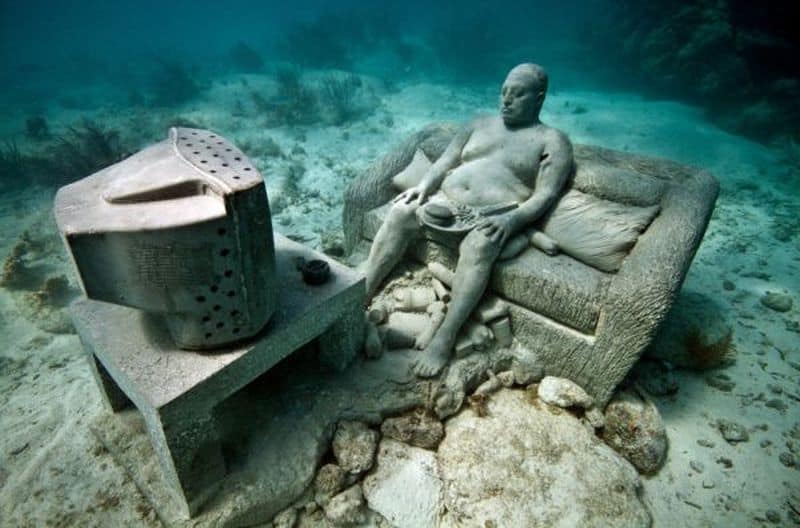This captivating underwater photograph captures a surreal, stone tableau set against a gradient backdrop that shifts from dark blue to a lighter bluish-turquoise. It features a life-size, stone sculpture of an overweight, bald man, sitting shirtless and pantsless on a stone couch with stone pillows. The man appears engrossed in watching an old-school, stone CRT television set perched on a solid, square-shaped stone coffee table in front of him. His hands rest naturally on his knees, and he balances a stone plate on his lap, which holds what looks like a stone hamburger. The underwater scene is textured with a sandy, rocky seabed interspersed with plants, lending an eerie yet realistic ambiance. The meticulous details, such as the man's big belly and a familiar domestic setup, evoke a sense of everyday life, frozen and submerged in a dreamlike aquatic environment.